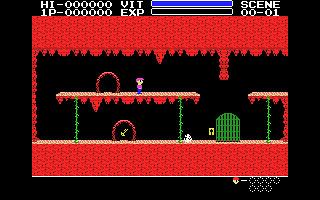This screen capture depicts a scene from an early vintage video game. Central to the image is a character donning a purple shirt, blue pants, and sporting a brown bowl-cut hairstyle, standing on an elevated platform. This platform is supported by two green poles. The background is stark black, emphasizing the simplicity of the game's visuals. Behind the character, there is a hoop-like structure, adding a layer of mystique to the scene. Below the platform, another hoop-like object is visible, containing a central element that is not clearly discernible. The frame surrounding the image is a striking red, which contrasts with the otherwise dark and minimalist background. Positioned between a gap in the platform, there is a green door, while a long, stalactite-shaped protrusion hangs down over this gap. At the top of the screen, various initials, zeros, and scenes are displayed in white text, characteristic of game score or player information in vintage gaming interfaces.